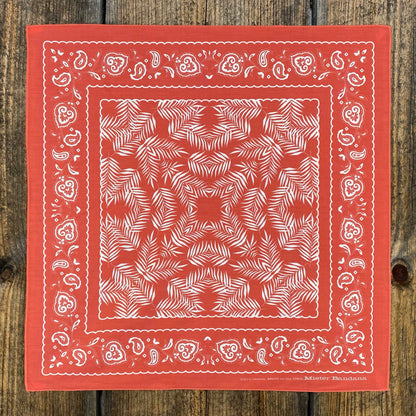The image showcases a vibrant, red square bandana laid flat against a backdrop of distressed medium oak wooden flooring. The fabric is meticulously decorated with intricate white patterns. Surrounding the bandana's edges is a scalloped border comprised of delicate, squiggly lines. Within this border are abstract symbols that resemble hearts, drops, or pear shapes, enhancing the decorative appeal. Progressing inward, two more scalloped borders frame the design, converging towards a central, symmetric pattern. This centerpiece features what seems to be a burst of fractal or ice crystal-like shapes, radiating outward like symmetrical pine branches or palm fronds. The bandana's artful design, reminiscent of paisley and traditional Mexican-style fabric, creates a harmonious and detailed visual, making it a striking piece of textile craftsmanship. There is no text on the fabric, emphasizing its purely decorative nature.